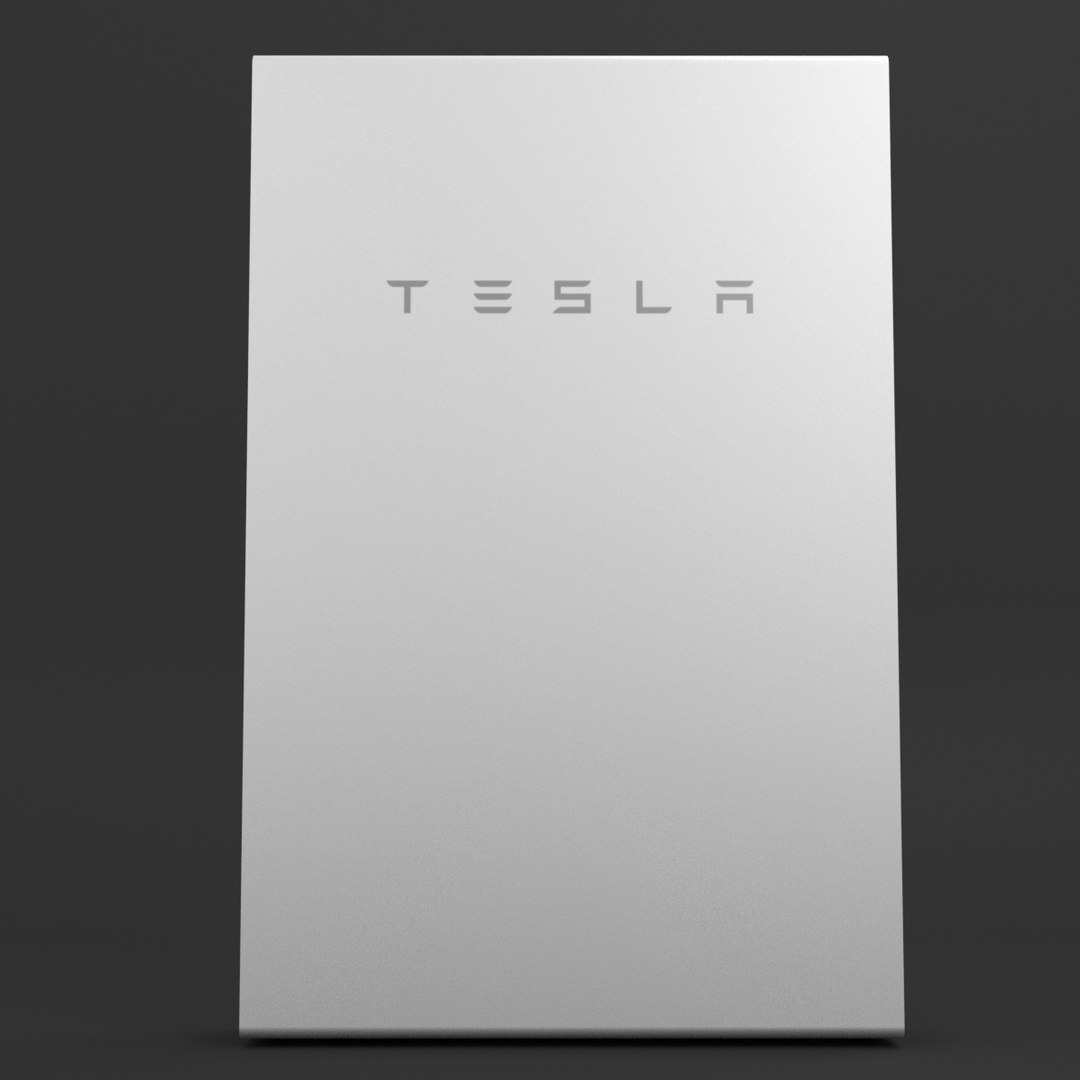This image, potentially designed for a Tesla-related webpage, features an intricately detailed metallic column prominently positioned against a gradient background that transitions from black at the top to dark gray at the bottom. The column, with a sleek and smooth surface, showcases the iconic Tesla logo at the top center, rendered in a distinctive stylized font. A subtle highlight on the column's upper right side suggests a light source positioned just off-camera, adding dimension and depth to the scene. The image is formatted in a 4x3 aspect ratio, indicative of web embedding rather than full-page display. The minimalist composition, devoid of any additional contextual elements, underscores the column's significance and likely aligns with Tesla's brand aesthetics typically featured on their digital platforms.